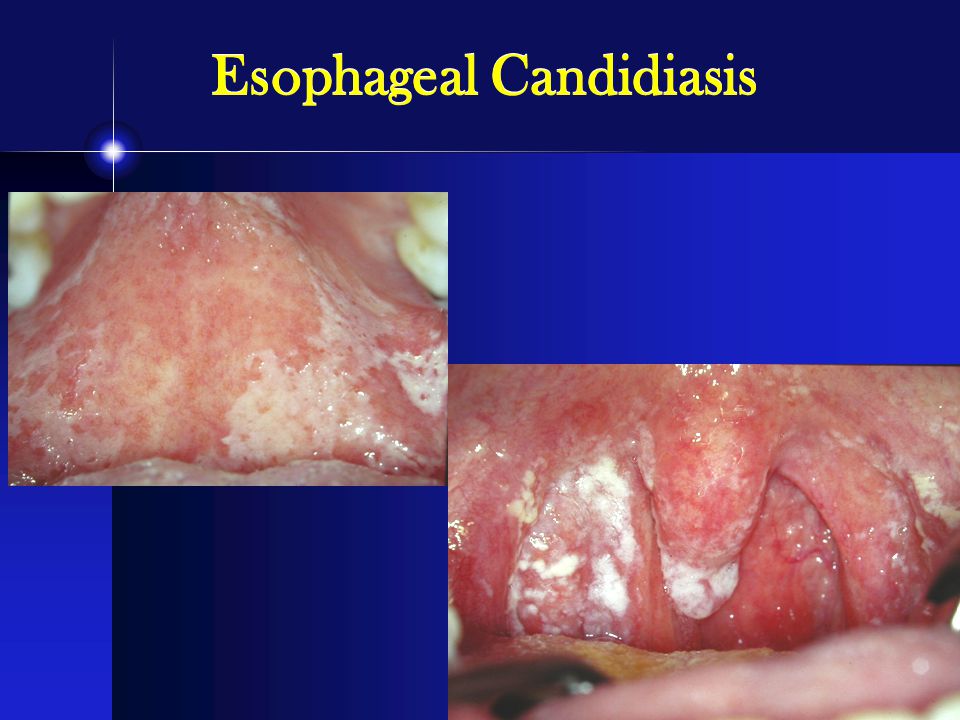The image is a slide from a PowerPoint presentation on esophageal candidiasis. At the top center of the slide, in gold (or possibly yellow) letters on a dark blue header, is the title "Esophageal Candidiasis." Below the title, to the left side, there is a glowing white ball of light marking the separation between the header and the content. The slide features two images depicting the biological condition. The left image shows the interior of the esophagus with a slight white appearance due to Candida infection. The lower right image is more graphic, displaying a heavily infected esophagus with significant white patches amidst visible red blood vessels, indicating severe candida overgrowth. The background of the slide is blue, enhancing the visibility of the images and text. Overall, the images emphasize the presence of white fungal film associated with esophageal candidiasis within the mouth and esophagus.